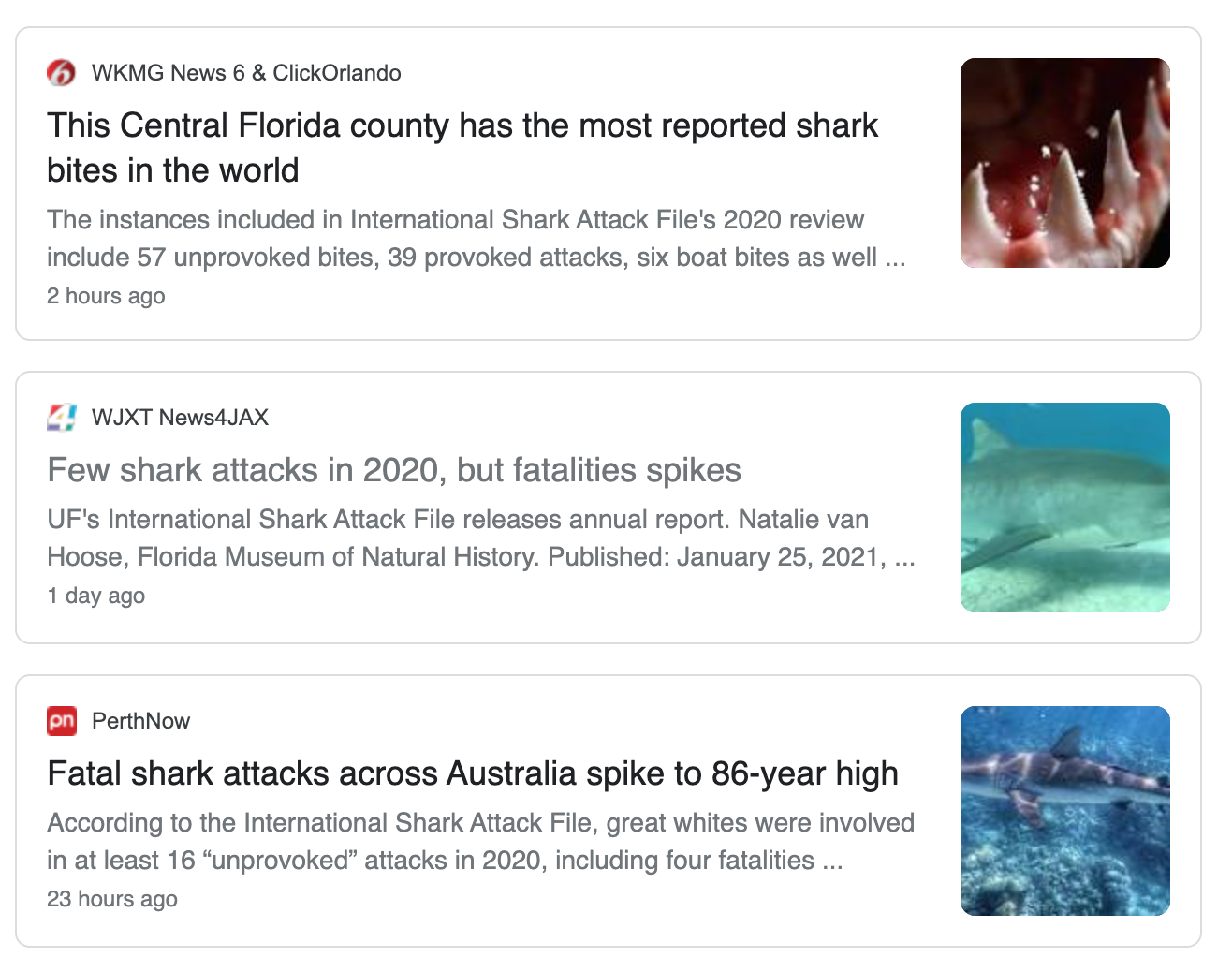The image is a collage of screenshots from various news articles, arranged vertically. The top article is from WKMG News 6 in Orlando, identified by its logo featuring a red circle with a number six in white font. The headline reads, "This Central Florida County has the most reported shark bites in the world," and is accompanied by a gruesome image of a shark's mouth with sharp, white teeth and blood. Beneath it, explanatory blurbs provide further details.

The middle article is from WJXT News 4 Jax, featuring their logo with a number four in a box. Its headline states, "Few shark attacks in 2020 but fatality spikes." This article includes an image of a gray shark, characterized by its white belly and dorsal fin, swimming underwater in clear, blue Caribbean-like waters.

The bottom article is from Perth Now, marked by a red square with white lettering in its logo. The headline announces, "Fatal shark attacks across Australia spiked to 86 year high." This article also includes an underwater image of a shark, which appears to be of a similar species swimming in blue waters, akin to the shark in the middle article.